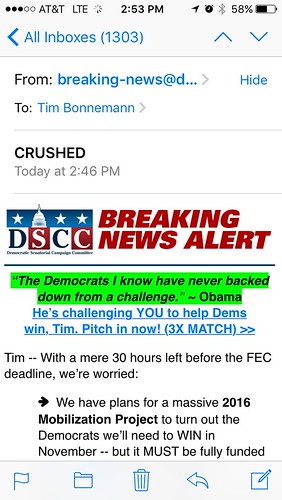**Descriptive Caption:**

A detailed screenshot of an email inbox on a mobile device:

At the top of the screen, there are five circular icons on the right side; three are solid black and two are black outlined in white. The status bar displays the AT&T LTE signal, a loading icon resembling a sun, the time "2:53 PM," a location or send icon, an activated alarm clock, the Bluetooth logo, and a battery indicator at 58%.

In blue font, there is a left-pointing arrow labeled "All Inboxes" with the number "1303" in parentheses. Below are navigation arrows to move between emails. The email header includes "From" in black font followed by "Breaking News at" with a partially obscured handle "D dot dot dot" in blue font. The "To" field shows "10 Bonneman" in blue font. The subject of the email is "Crushed," received today at "2:46 PM."

The body of the email features a "DSCC Breaking News Alert" banner with the US Capitol building icon in blue, white, and red colors. The text "Breaking News Alert" is highlighted in red. A green-highlighted quote from Obama reads, “Democrats I know have never backed down from a challenge.” The email urges, "He's pitching you to help Dems. When Tim pitch in now," with an emphasis on a "three times match" offer in blue font.

The message continues: "Tim, with a mere 30 hours left in the FEC deadline, we're worried. We have plans for a massive 2016 mobilization project to turn the Democrats, and we need a win in November. We must be fully funded."

Icons at the bottom of the screen show options for flagging, moving to a folder, deleting the email, and navigating back and forth.